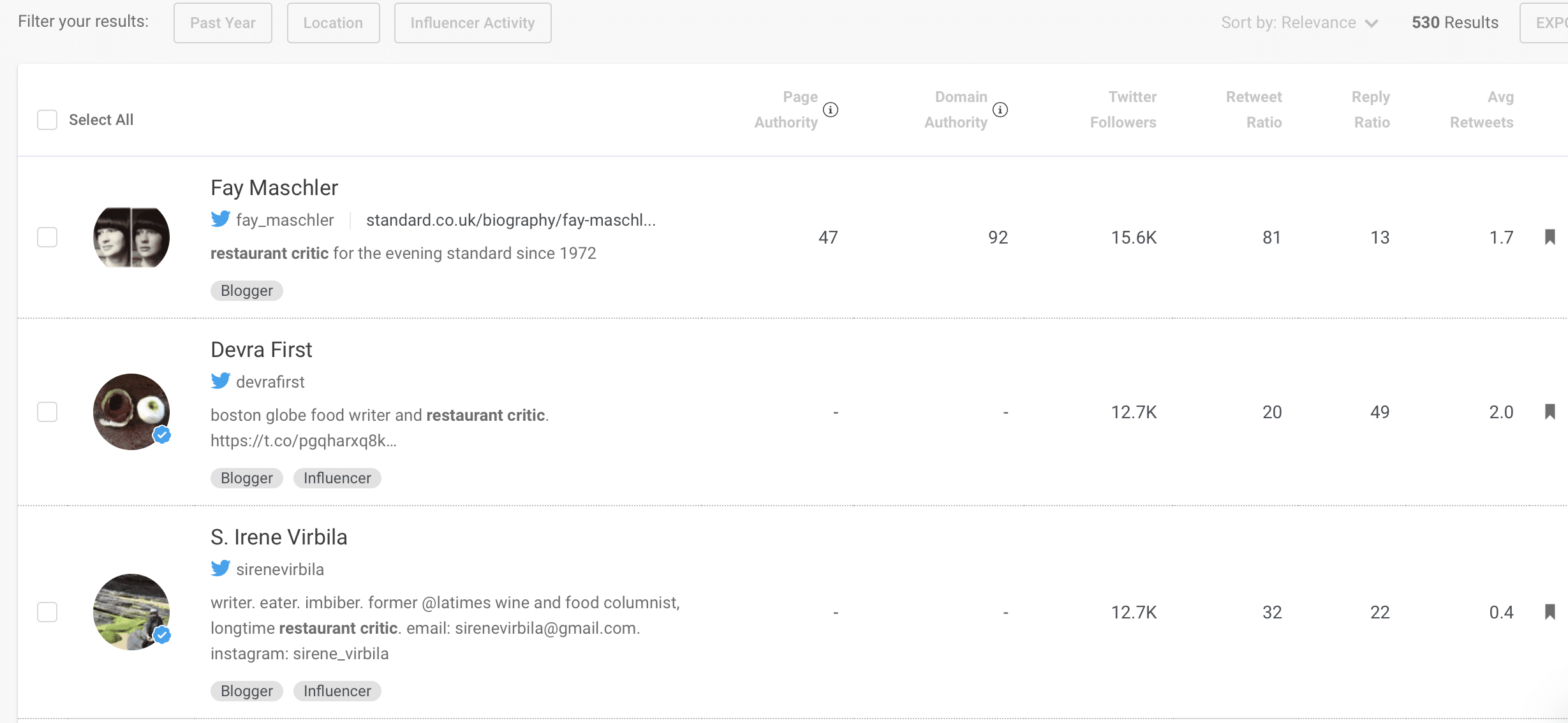In this image, we see a webpage featuring a list of bloggers and influencers, displayed on a background with a light smoke-gray color that is prominent at the top and left sides, with a slight hint at the bottom. In the upper-left corner of the image, there are filtering options that read "Filter your results: Past Year, Location, and Influencer Activity." On the right side, it says "Sort by relevance" followed by "530 results."

Below this, there is a white box that includes selection checkboxes on the left to "select all" and individual checkboxes next to each person's name. The names listed are Faye Manchler, Debra First, and S. Irene Verbilla. All three are identified with Twitter accounts, and Faye Manchler is noted as just a blogger, while Debra First and S. Irene Verbilla are both bloggers and influencers. 

To the right, the page displays authority metrics including "Main Authority," "Twitter Followers," "Retweet Ratio," "Reply Ratio," and "Average Retweets."